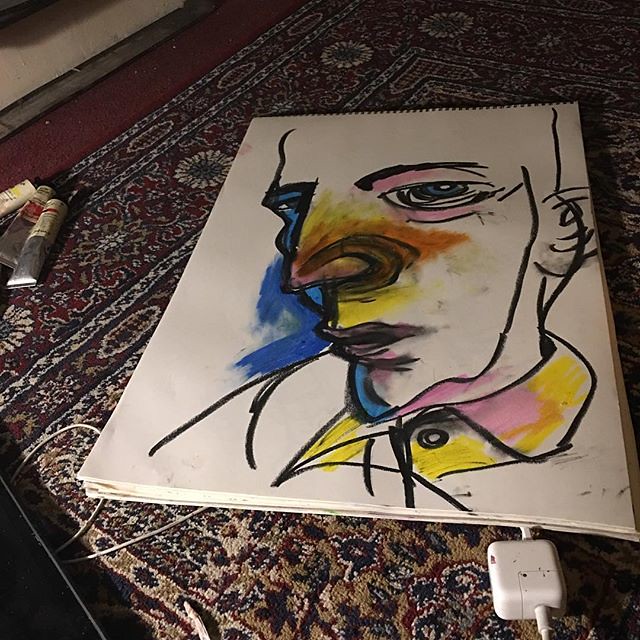The image showcases a vivid colored sketch painted on a large white poster board paper, which is part of a spiral-bound poster board binder. The artwork features a male subject with fair skin. His left ear is prominently larger and extends outward from his head. The eyes are strikingly blue, with a subtle pink hue around the eyelids. His nose is sharply defined and adorned with an intriguing blend of yellow, orange, and brown tones, complemented by a hint of pink at the tip. His thin lips are slightly pink, matching the delicate coloring around his eyes. The subject is depicted wearing a shirt, with a collar that has been painted in a distinct pink color. This detailed and expressive portrait captures the viewer's attention with its vibrant palette and unique artistic style.